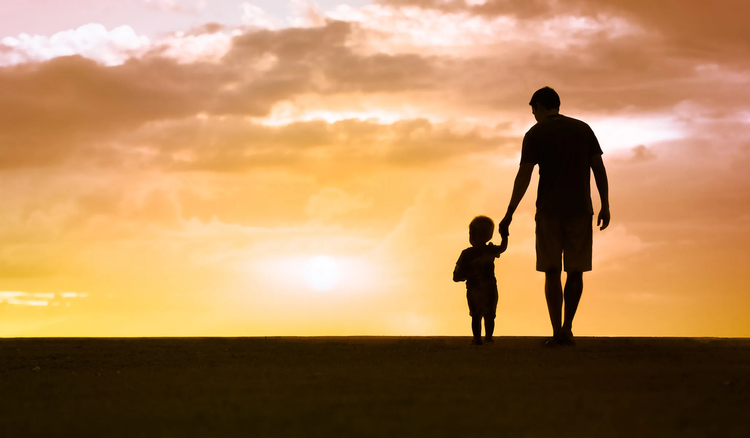The image captures a poignant scene of a man and a young child, possibly a few years old, walking hand in hand against a stunning sunset backdrop. The silhouettes of the man and child, both dressed in shorts and t-shirts, stand out in stark black against the vivid colors of the sky. The man is slightly leaning over, tenderly holding the child's left hand with his right. They appear to be walking on a flat, black surface that merges seamlessly with their dark silhouettes. The sunset dominates the background, with a dazzling array of yellow, orange, and pink hues illuminating the clouds, casting a serene glow across the scene. The sun is positioned low in the sky, near the bottom of the frame, enhancing the dramatic effect of the silhouettes. The peaceful and intimate interaction between the man and the child is the focal point, framed beautifully by the expansive, colorful sky.